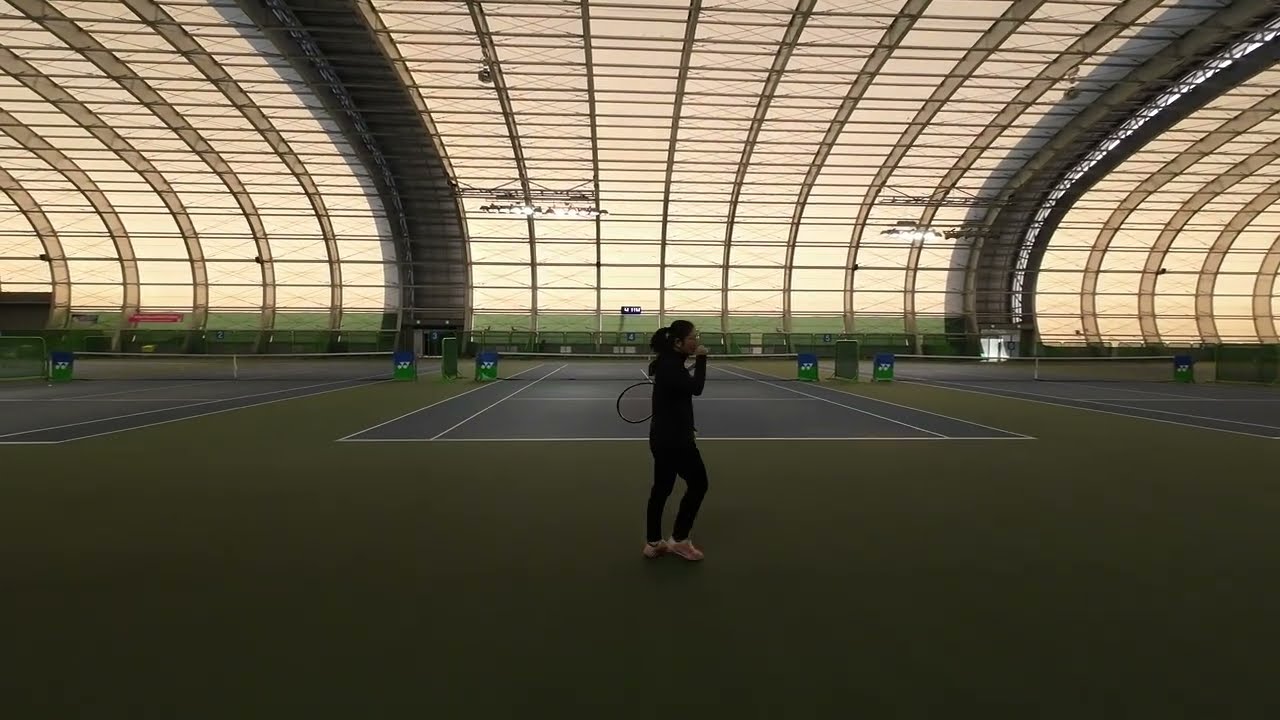This detailed photograph captures the interior of a vast indoor sports facility, clearly designed for racket sports, featuring three visible badminton courts. The center court is fully visible, displaying a gray surface with precise white lines, while the adjacent courts are partially obscured. Surrounding the courts, the ground area is distinctly green. Prominently positioned in front of the middle court is a woman clad in a black dress, holding a badminton racket and facing towards the right. The arena's roof is architecturally striking, with its curved structure composed of cream-colored glass panels, from which several lights are suspended, contributing to the interior illumination. Despite the spaciousness and well-lit design, the facility has a somewhat subdued lighting ambiance, suggesting reliance on external light sources for optimal visibility. Additionally, green stands are situated nearby, potentially for storing balls and water.